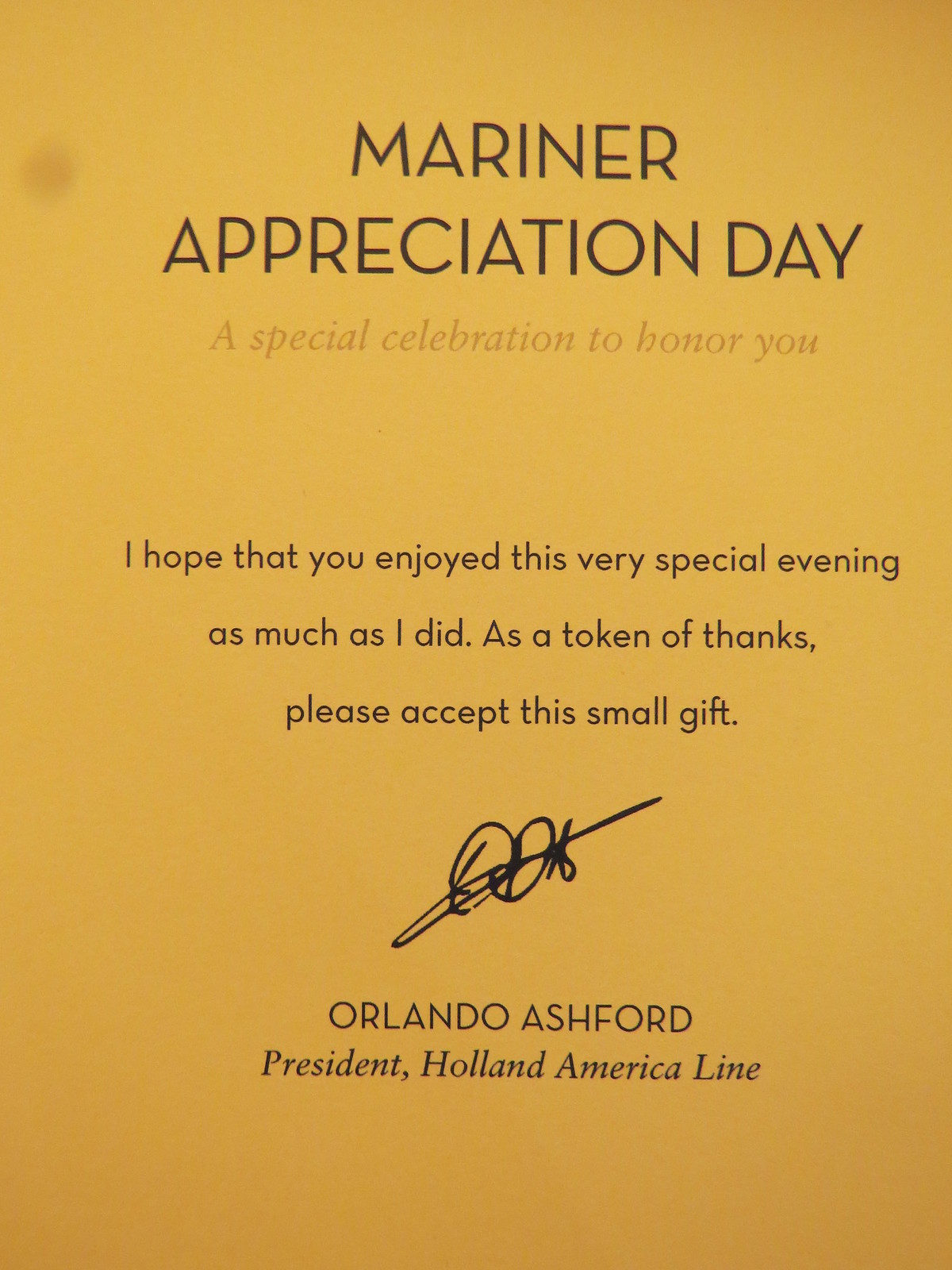This is a photograph of a flyer from a Mariner Appreciation Day event by Holland America Line. The flyer, approximately three by five inches in size, is a yellowish-gold color with darker gold and light brown prints. The main heading, "Mariner Appreciation Day," is prominently displayed in large, capitalized font. Below it, in a cursive-like text, it reads, "A special celebration to honor you," in a lighter shade, making it somewhat hard to read. The subsequent text, in regular black font, says, "I hope that you enjoyed this very special evening as much as I did. As a token of thanks, please accept this small gift." 

The document appears aged and has a smudge in the top left corner. It's signed at the bottom by Orlando Ashford, the President of Holland America Line, with his signature appearing somewhat messy, almost like a doctor's signature. The flyer was likely a personalized certificate accompanying a gift given to passengers, celebrating their appreciation day. There are no specific details such as date, location, or time mentioned on the flyer.